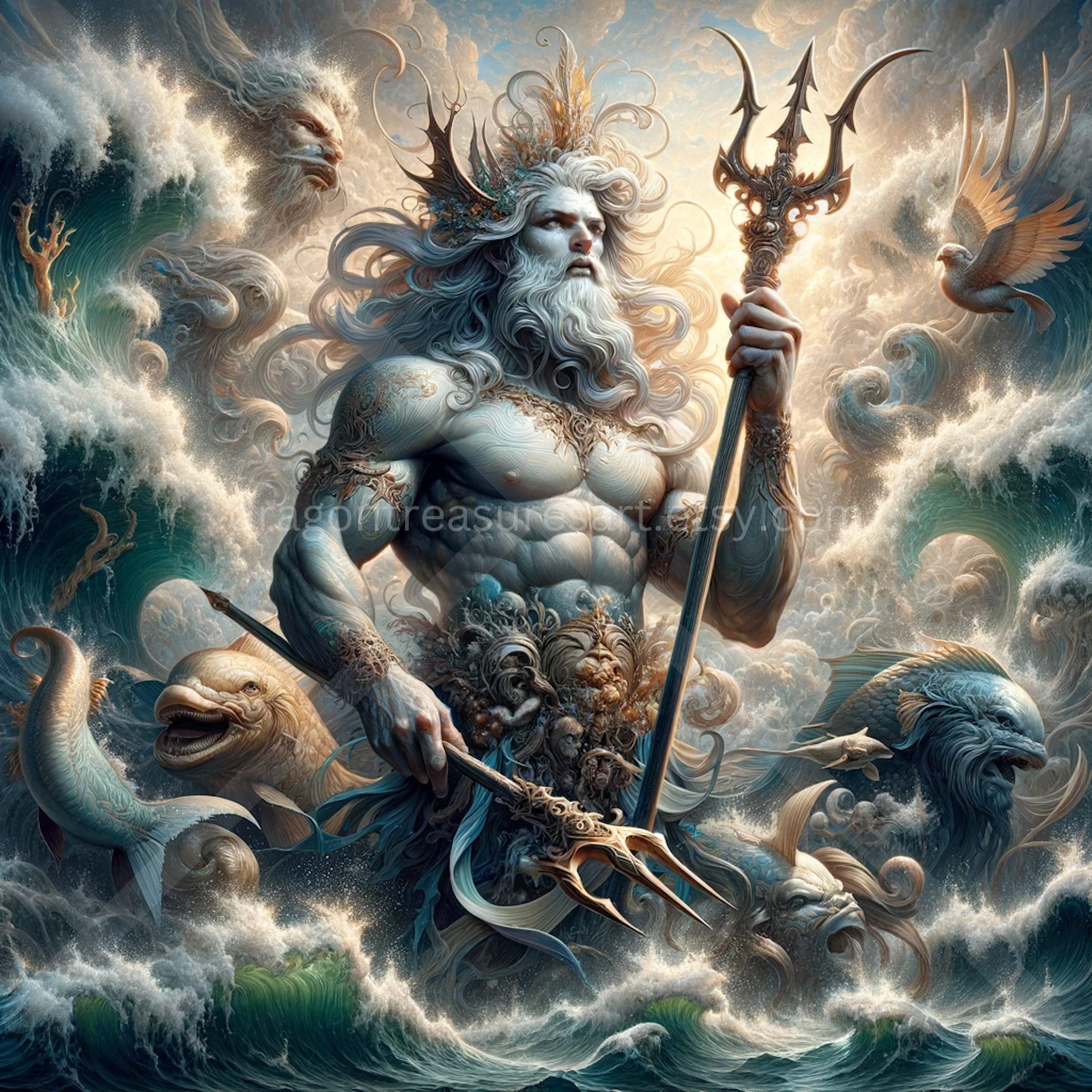This highly detailed digital pixel art image features a vigorous, extremely muscular, late middle-aged Poseidon occupying the center of the frame. He is vividly depicted with wind-tossed long white hair and a matching beard, adorned with an elaborate golden crown. Poseidon's light blue skin glistens as he holds two tridents—one shorter than the other. His abdomen is shielded by an intricately scrolled metal plate, matching his ornamental wrist, arm bands, and neck band, along with a belt inlaid with golden shells and coral. 

The stormy sky serves as a dramatic backdrop, with ocean waves rising majestically on either side of him. The scene is teeming with life as various sea creatures like dolphins and fish, as well as flying birds, surround Poseidon. Interestingly, there's another human face in the clouds—possibly representing Zeus or one of the winds—peering down upon the ocean god. The inscription "ragontreasureart.etsy.com" is emblazoned across the center, adding an artistic touch to this captivating portrayal of Poseidon emerging from the tumultuous sea.